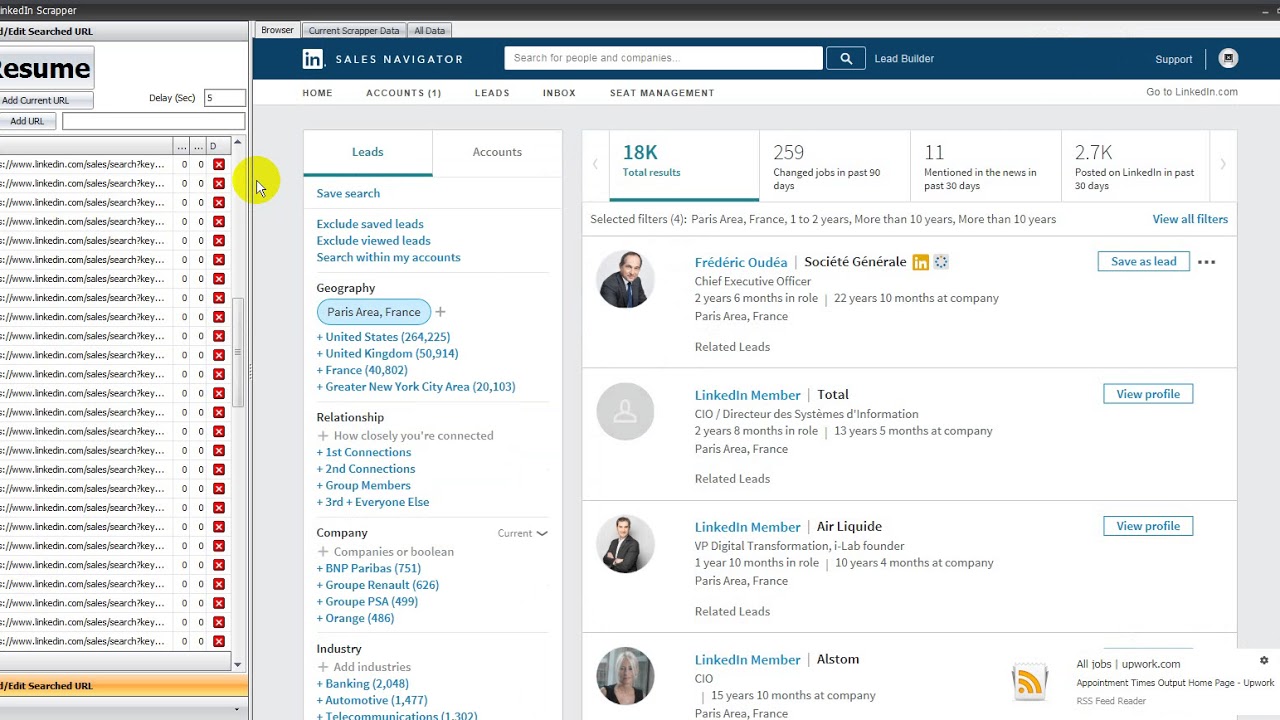The image depicts a detailed view of a website interface, likely showcasing search results from a sales navigation platform. 

The main layout consists of a pale grey background with white information boxes overlaying it. At the very top, there is a dark grey navigation bar. On the left-hand side of the main body, the word "Resume" or "Résumé" appears, followed by a sequence of search results numbered from 1 to 26.

On the right-hand side of the screen, there's a distinct blue navigation bar at the top featuring an 'IN' icon in a white square, denoting LinkedIn's "Sales Navigator". Next to the icon, it says "Sales Navigator". The navigation bar also includes a search bar and options for "Support" and "Profile".

Other available navigation buttons include "Home", "Accounts", "Leads", "Inbox", and "Seat Management". Below the navigation bar on the left-hand side, there's a white box titled "Leads and Accounts". The user is currently on the "Leads" tab, with additional options to save the search, exclude saved leads, exclude viewed leads, and search within "My Accounts". 

The search is focused on "Geography" with the "Paris Area, France" selected. Additional filter options include "Relationship", "Company", and "Industry".

To the right within the white information box, there are 18,000 total search results displayed. Notably, 259 individuals have changed jobs in the past 30 days, there have been 11 news mentions in the same period, and 2.7 thousand posts on LinkedIn in the past 30 days.

Beneath this summary, the user can see four specific results, each featuring a profile picture on the left, the individual's name, and some brief information about them.